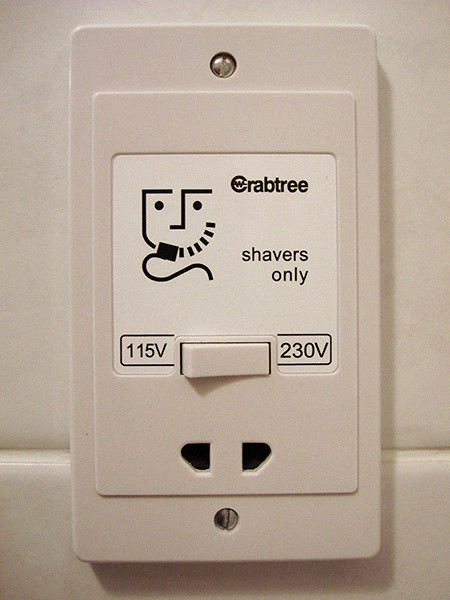This image depicts a cream-colored, rectangular electrical socket mounted on a wall with ceramic tiles and white grout. The socket appears to be designed for international use, allowing for voltage selection between 115 volts and 230 volts via a small flip switch. Below the switch, there are two plug holes that resemble a peculiar socket, likely intended for specific devices. The center of the socket features the brand name "Crabtree" and an illustration of a face with noticeable eyebrows, eyes, nose, and chin. The label above the plug holes reads "shavers only," indicating its exclusive use for electric shavers. The image suggests the socket is positioned in a bathroom or similar setting due to the tiled backdrop.